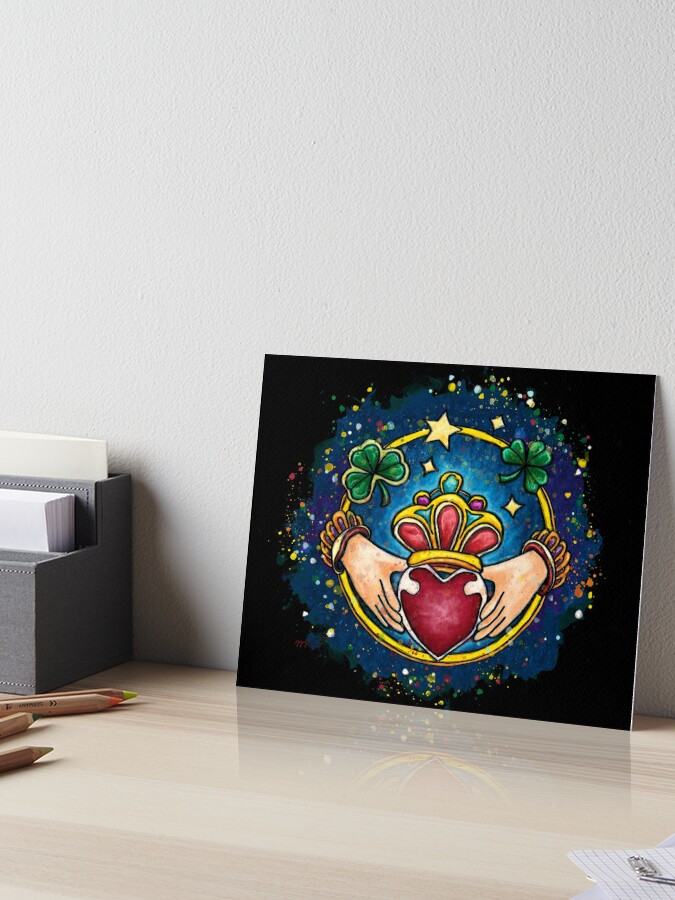This indoor photograph showcases a charming, handmade piece of art displayed on a shiny light brown desk, leaning against a white wall. On the left side of the desk are several beige colored pencils with various colored tips, likely utilized in creating the artwork. In front of these pencils is a gray rectangular paper organizer holding some white papers or envelopes. 

The art itself is a striking, rectangular painting depicting a vivid red heart adorned with a crown at its peak. Two white, unconnected hands reach down to hold the heart, both hands featuring beaded bracelets. Encircling this central motif is a golden ring with green clovers, sometimes described as four-leaf and other times three-leaf, floating at the top, along with stars dotting the area above. The background behind the ring resembles a dark blue, space-like sky filled with colorful speckles of yellow, blue, and red, transitioning to a completely black border around the edge. The painting is created in a distinct, cartoony style, adding to its whimsical charm.